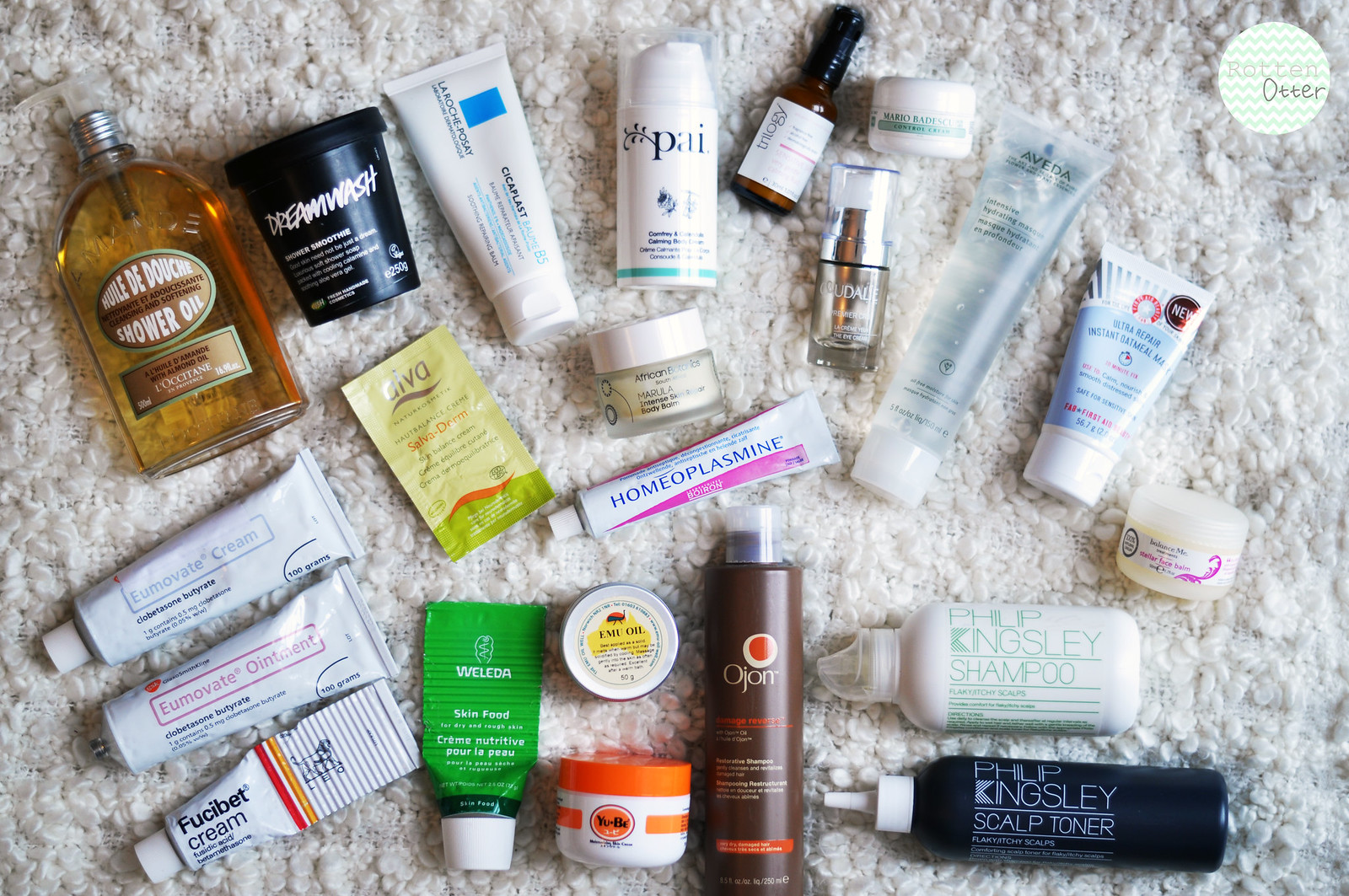This image showcases an aesthetically arranged collection of 22 beauty products displayed on a pristine white fur carpet. Each item is meticulously positioned, creating a visually appealing and elegant presentation. In the top right corner, a distinctive green and white circular logo bearing the name "Rotten Otter" adds a touch of brand identity to the scene. 

The products include a variety of skincare and haircare essentials with names such as Shower Oil, Dream Wash, Fusibet Cream, You Motivate Ointment, You Motivate Cream, Salvaderm, Weleda Skin Food, Homoeoplasmine, Avéda, and Philip Kingsley Scalp Toner. Other notable items are Philip Kingsley Shampoo, Ozone, Emu Oil, UBC, African Pride, and brands or labels that seem to read Sisa, Plas, La Roche, and Rose. The assortment displays a diverse range, suggesting a well-rounded beauty regimen. 

Overall, the composition not only highlights the beauty products' branding but also emphasizes their luxurious and pampering nature, perfectly suited for any beauty enthusiast.